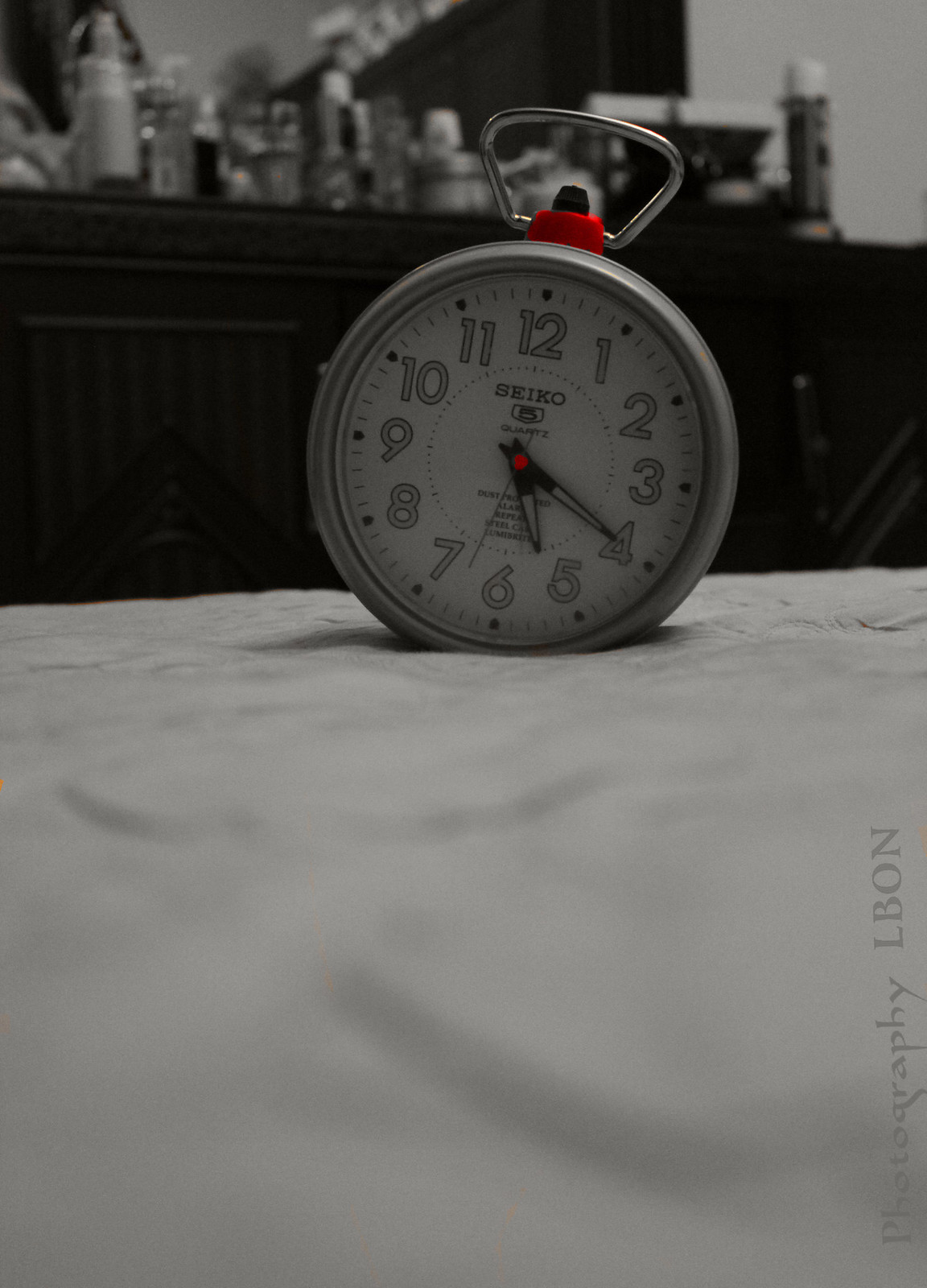In this softly lit, gray-toned interior, an elegant Seiko alarm clock sits on a neatly made bed, its legless form slightly tilting to the right. The clock, set at 5:20, features glow-in-the-dark hour and minute hands, and distinct numbers 1 through 12. In the background, a dark wood dresser is visible, cluttered with a variety of hygienic products, including bottles, cans, and sprays, while a mirror attached to the dresser can be faintly seen in the distance. The bedding on the bed is a matching soft gray, enhancing the serene ambiance of the room.